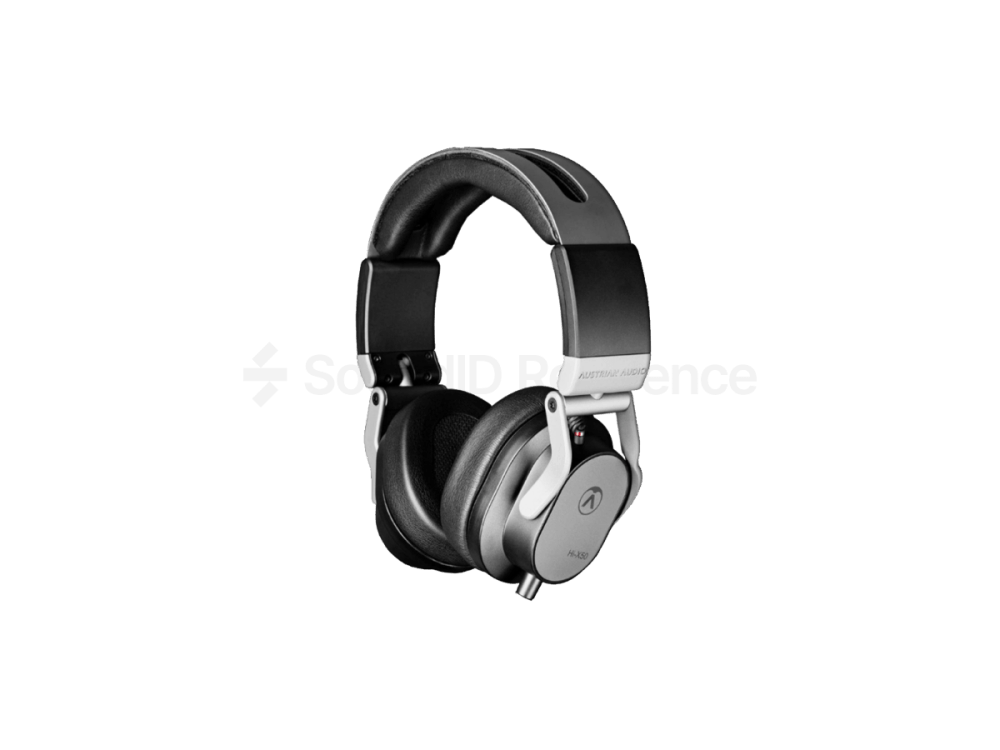The image showcases a professional pair of black and gray headphones, set against a pure white background. The headphones have a distinctly blocky and somewhat angular design, featuring well-padded, black cushioned earpieces and additional padding along the top arch for enhanced comfort. The top arch itself is dark gray, and beneath it lies a dark black pad. The black cups of the headphones have flat faces with an upside-down V logo encircled by a thin light gray ring. Additionally, the headphones feature a black curved rectangular piece that connects to a white small rectangle, which is attached to a white rod by two white boomerang-shaped pieces.

A watermark with text and an S-shaped logo made of three light gray rectangles is partially visible on the image, with the letters "S-O" appearing to the left of the headphones, "I-D" obscured by the headphones, and "E-N-C-E" visible to the right. The insignia HI-X50 on the earpiece likely denotes the model number. A small red light, possibly indicating the on-off status, provides the only splash of color. The trademark and watermark suggest the image belongs to Australia Audio, barring any conflicting identifications.